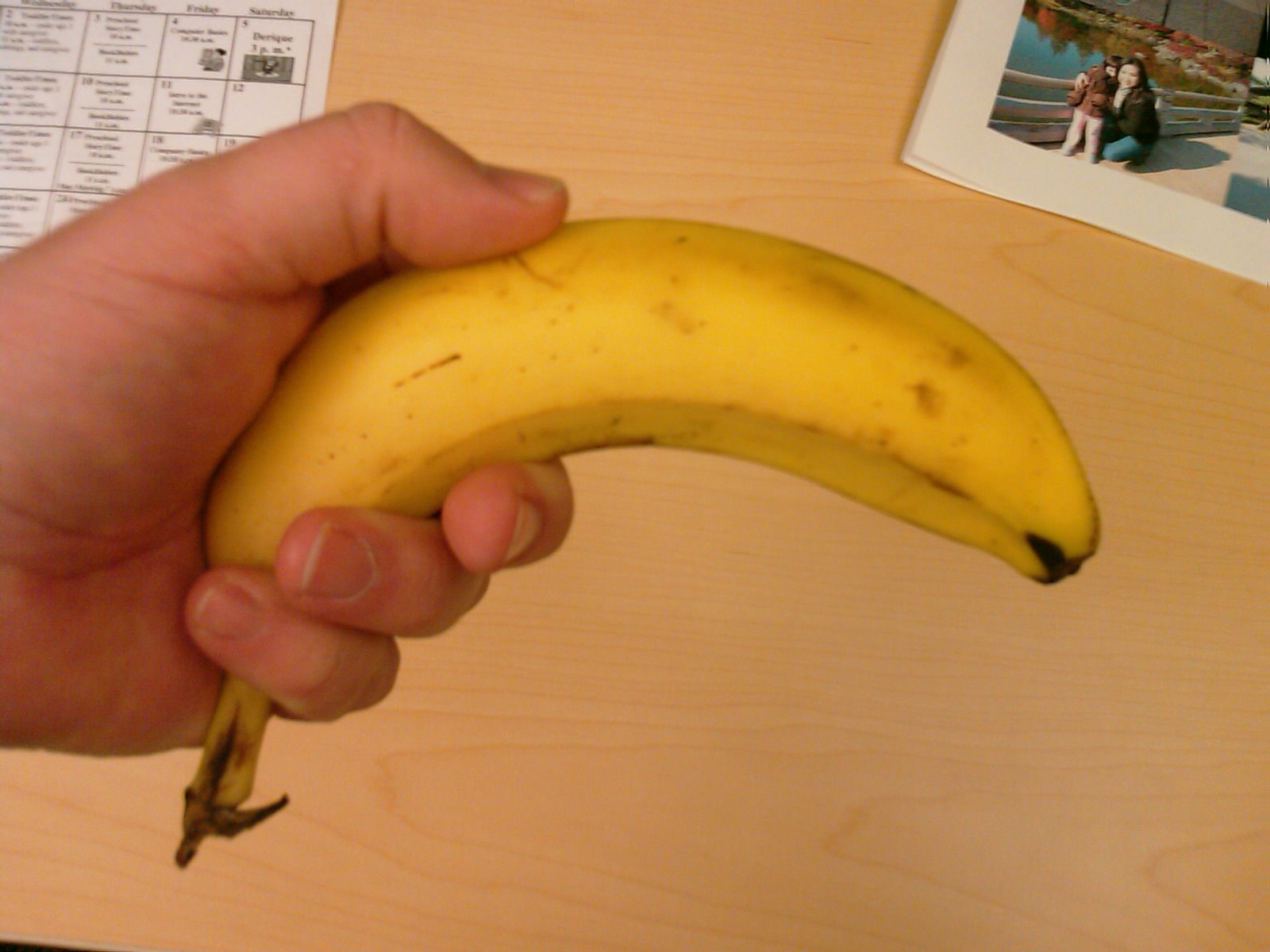A close-up captures a man's hand holding a medium-sized, ripe banana. The banana is bright yellow with several dark brown spots and flecks, indicating its ripeness. The scene is set against a wooden tabletop, where a planner lies open. The planner displays the days of the week across the top, with various dates, text, and images filling the individual daily squares. In the upper right corner of the image, there's a photograph featuring a woman and a child posing beside a small pond. The detailed setup and the ripe banana held in the man's hand create an intriguing point of focus against the organized backdrop of the planner and the personal touch of the photograph.